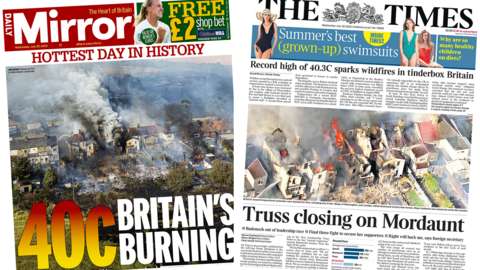This image features two newspapers side by side. The newspaper on the left is the *Daily Mirror*, and the one on the right is the *Times*, a London-based newspaper. The newspapers appear to be tabloid-size; however, the image of the *Times* on the right is cut off at the bottom, leaving the possibility that it might be a broadsheet.

The *Daily Mirror* on the left showcases a dramatic aerial view of a burning house with smoke billowing out of the large structure. Overlaid at the bottom of this photo is a graphic with yellow and dark red colors indicating a temperature of 40°C (40 Celsius). At the bottom of the image, a bold white twin stack headline reads, "Britain's Burning." Above the image, a red headline states, "Hottest Day in History."

The *Times* newspaper on the right appears to be from the same day. Just below the masthead, alongside an advertisement for swimsuits, is the headline, "Record high of 40.3°C sparks wildfires and tinderbox Britain." It also features an aerial view of burning homes, which might be the same scene depicted in the *Daily Mirror*. Below this image, another headline reads, "Trust closing on Mordaunt."

Both newspapers highlight the extreme heat and resulting wildfires, visually emphasizing the unprecedented weather conditions in Britain.